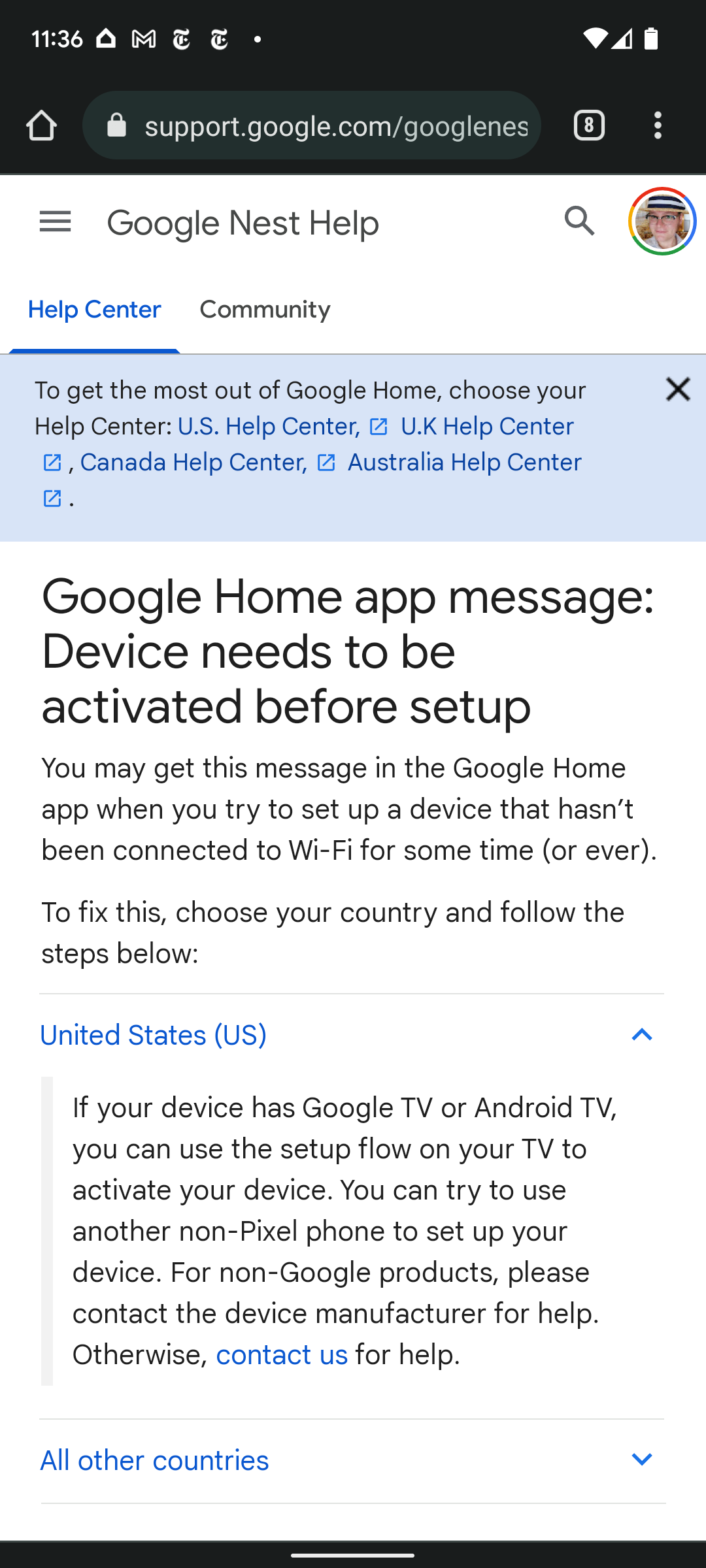A user is depicted in the image browsing the Google support website on a mobile phone, accessing the site via the Chrome browser. The specific URL visited is support.google.com, and the user is in the "Google Nest Help" section. The interface is divided into two primary sections: "Help Center" and "Community," with the user currently viewing the "Help Center." 

The displayed page contains a detailed guide titled "Google Home App Message: Device needs to be activated before setup." The message alerts users that they may encounter this notification in the Google Home App when attempting to set up a device that has either never been connected to Wi-Fi or hasn't been connected for a significant period. 

To resolve the issue, the guide instructs users to select their country and follow the ensuing steps. In this case, the country selected is the United States. The instructions note that for devices with Google TV or Android TV, users can employ the setup flow directly on their TVs to activate the device. It also suggests using an alternative non-Pixel phone for setup or contacting the device's manufacturer for non-Google products. A "Contact Us" link, highlighted in blue, directs users needing further assistance to Google support.

The layout of the page is clean with a white background and black text, maintaining Google’s typical minimalist design. The user's profile picture is visible; it features a young white male wearing a whimsical turn-of-the-century carnival hat, adding a touch of personality to the otherwise technical scene.